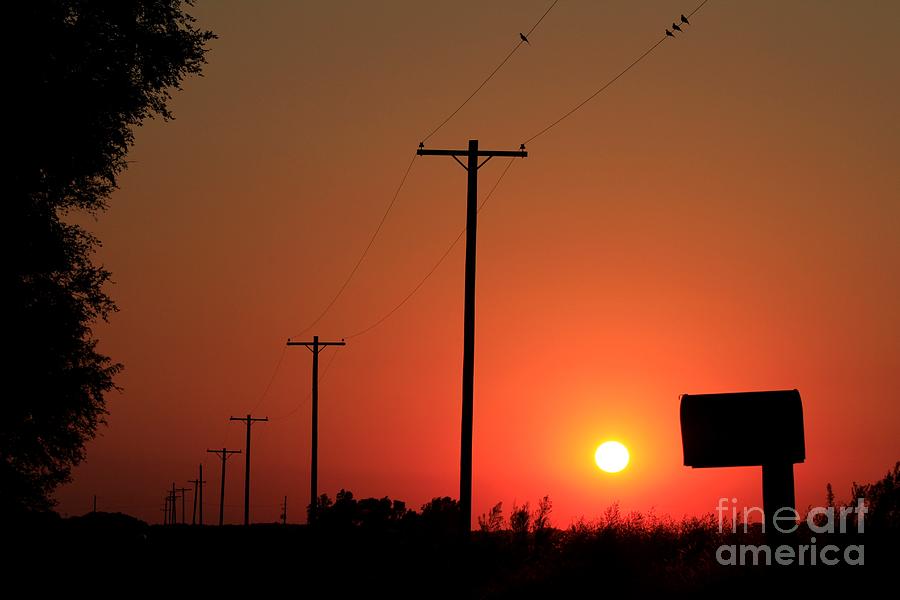This is a detailed sunset photograph captured in a rural area, with the sky painted in vibrant shades of orange and yellow. The low-hanging sun appears as a glowing yellow circle, casting an enchanting orange hue over the entire scene. In the foreground, a traditional mailbox stands beside a long, unseen road, indicating a serene countryside setting. Silhouetted against the radiant sky are T-shaped power line poles stretching into the horizon, with a striking arrangement of birds—three perched together on one wire and a solitary bird on another. The left side of the image is framed by the dark foliage of a tree, with its leaves reaching into the vibrant backdrop. Additionally, tufts of grass are silhouetted in the lower part of the photograph, enhancing the natural, untouched feel of the scene. In the bottom right corner, the text "Fine Art America" is subtly visible in white letters, adding a touch of elegance to the overall composition.